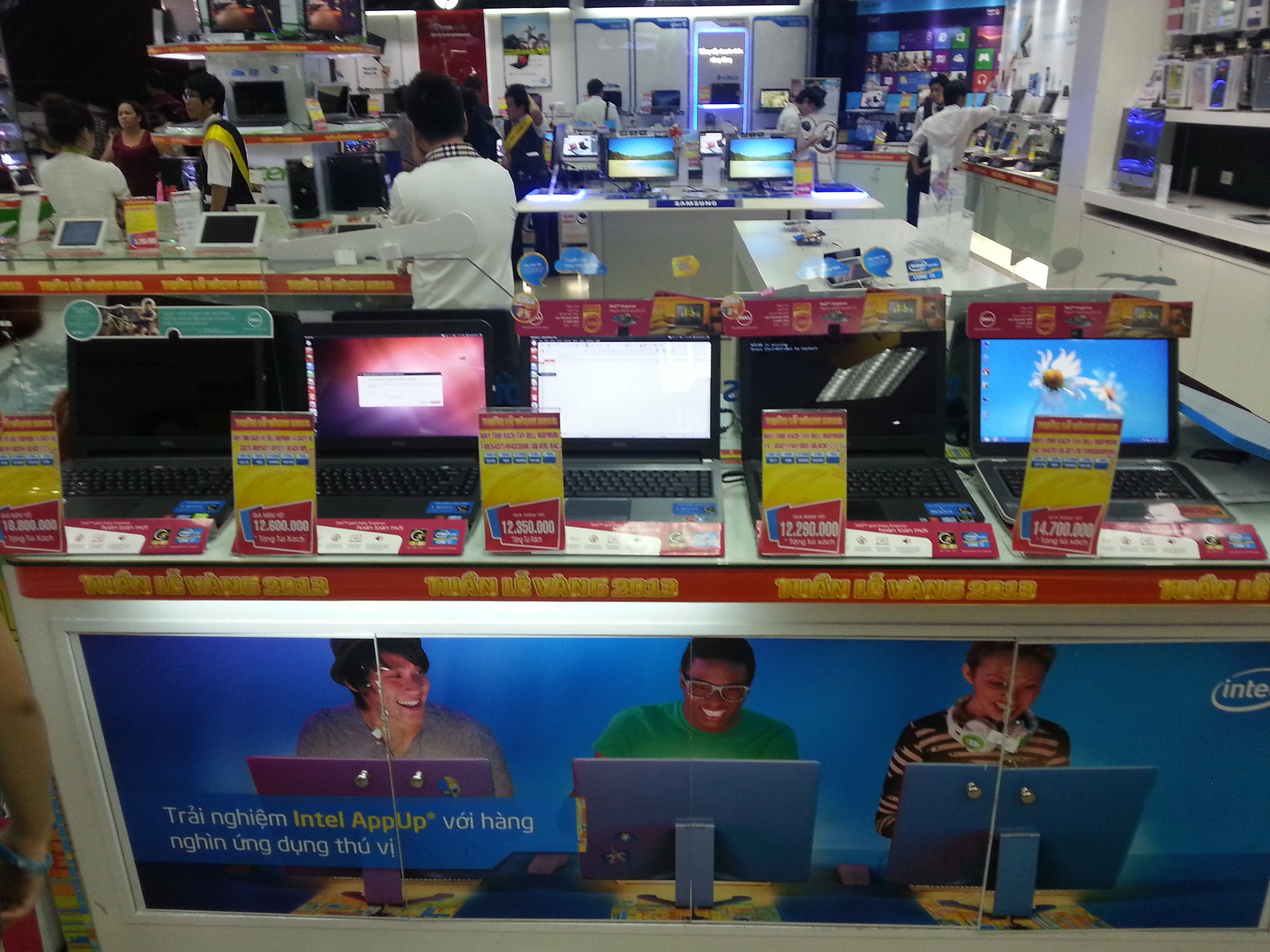The image portrays a bustling computer store, potentially located in Asia, possibly India or Vietnam, suggested by the appearance of the people and some of the language on advertisements. The main focus in the foreground is a row of five laptops displayed on a red ledge countertop, each with a yellow price card detailing specifications. Some laptops are powered on, showing various screens, while others are off. Beneath the laptops, an advertisement banner showcases three diverse individuals—an African-American boy in a green t-shirt with glasses, a white girl with short black hair wearing a black t-shirt with white stripes and headphones around her neck, and an Asian boy smiling in a gray t-shirt. They are all engaged with computer monitors, with the Intel logo and the text "Intel AppUp" prominently displayed. The store’s back area includes more tables laden with laptops, tablets, monitors, and other electronics. Several salesmen, identified by their white shirts, assist customers. The store is vibrant and full of activity, indicating a wide selection of tech products available for potential buyers to explore.